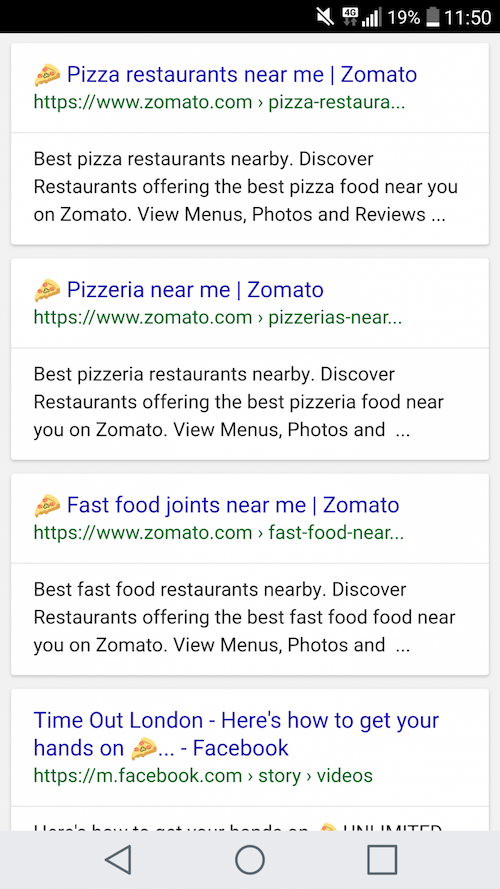In this image, we see a snapshot of a dining webpage, presumably viewed on a mobile device, with a focus on finding nearby restaurants. At the top of the page, there is a heading that states, "Pizza Restaurants Near Me - Zomato." Below this, a descriptive text reads, "Best pizza restaurants nearby. Discover restaurants offering the best pizza food near you on Zomato. View menus, photos, and reviews."

Beneath this initial section, there are four distinct rectangular blocks, each providing different restaurant search options. The first two blocks are nearly identical, featuring the same description about pizza restaurants, but with slightly different headings. The second block is titled, "Pizzeria Near Me," and maintains the same description as the first.

The third rectangular block diverges in its focus by stating, "Fast Food Joints Near Me - Zomato." Its accompanying description reads, "Best fast food restaurants nearby. Discover restaurants offering the best fast food near you on Zomato. View menus, photos." The text is abruptly cut off here.

The final block at the bottom of the page introduces a different context. It is branded "Time Out London" and includes the phrase, "Here's how to get your hands on..." followed by a small image of a piece of pizza. Below this image, there is an icon indicating a Facebook link.

Additionally, at the very top of the webpage, the device's status bar reveals a low battery at 19% and shows the current time as 11:50.